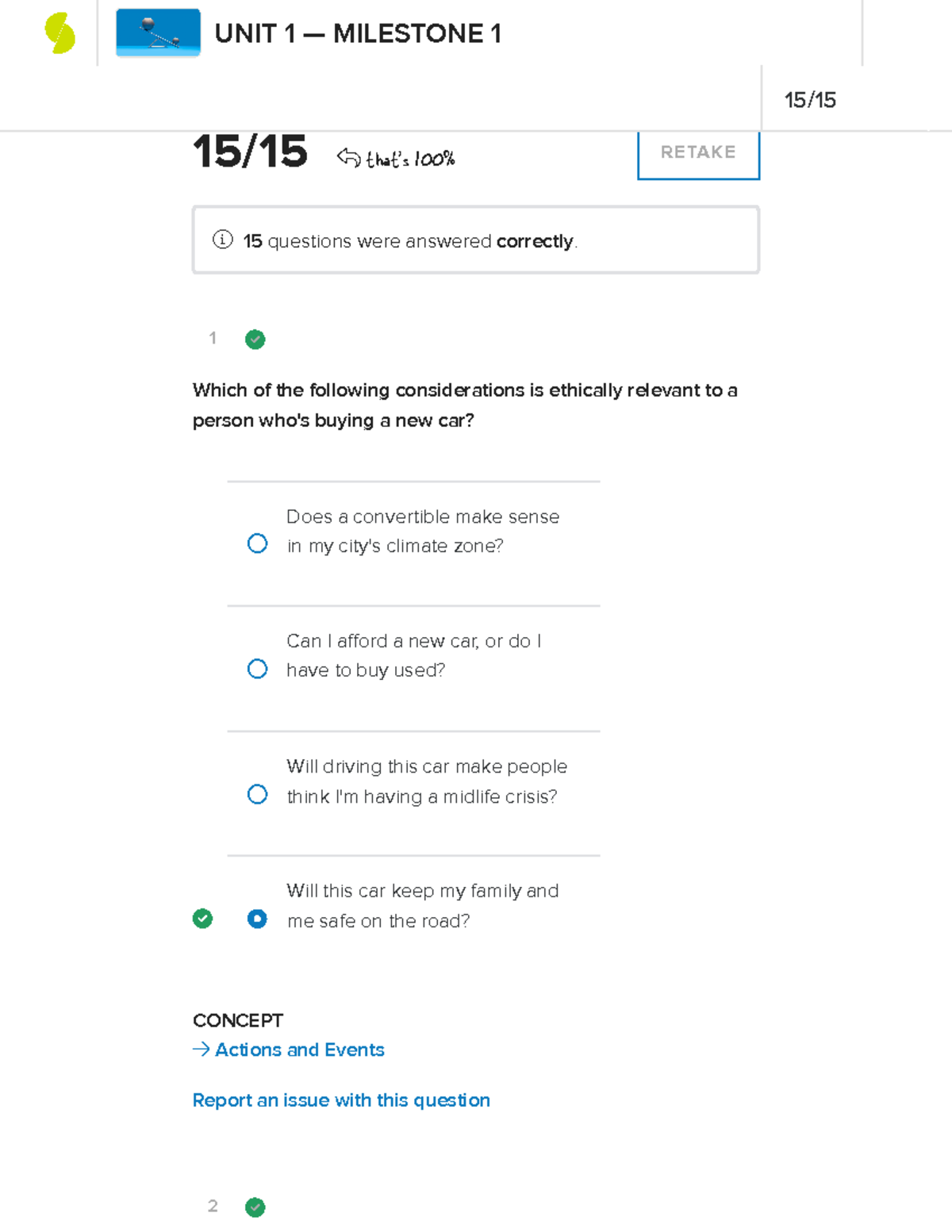The image features a predominantly white background. In the top left corner, there is an undefined gold symbol. To its right, there is a blue square with a gradient—dark blue at the top transitioning to light blue at the bottom. In black capital letters, to the right of the blue square, it reads "UNIT ONE MILESTONE ONE." Slightly below and to the right of this text, it says "15/15." A light gray line extends beneath this section.

Below the gray line, on the left side, in bold black letters larger than the other text, it reads "15/15." Next to this, there is smaller text with an arrow pointing toward it, which states, "That's 100%." To the right of this smaller text, there is a small box with the word "Retake" centered in black text.

Underneath, there is a light gray rectangle containing the following text in black: "15 questions were answered correctly." Below this is a small green circle, followed by black text that reads, "Which of the following considerations is ethically relevant to a person who's buying a new car?" The image also shows four options listed below this question, with the bottom option being selected.